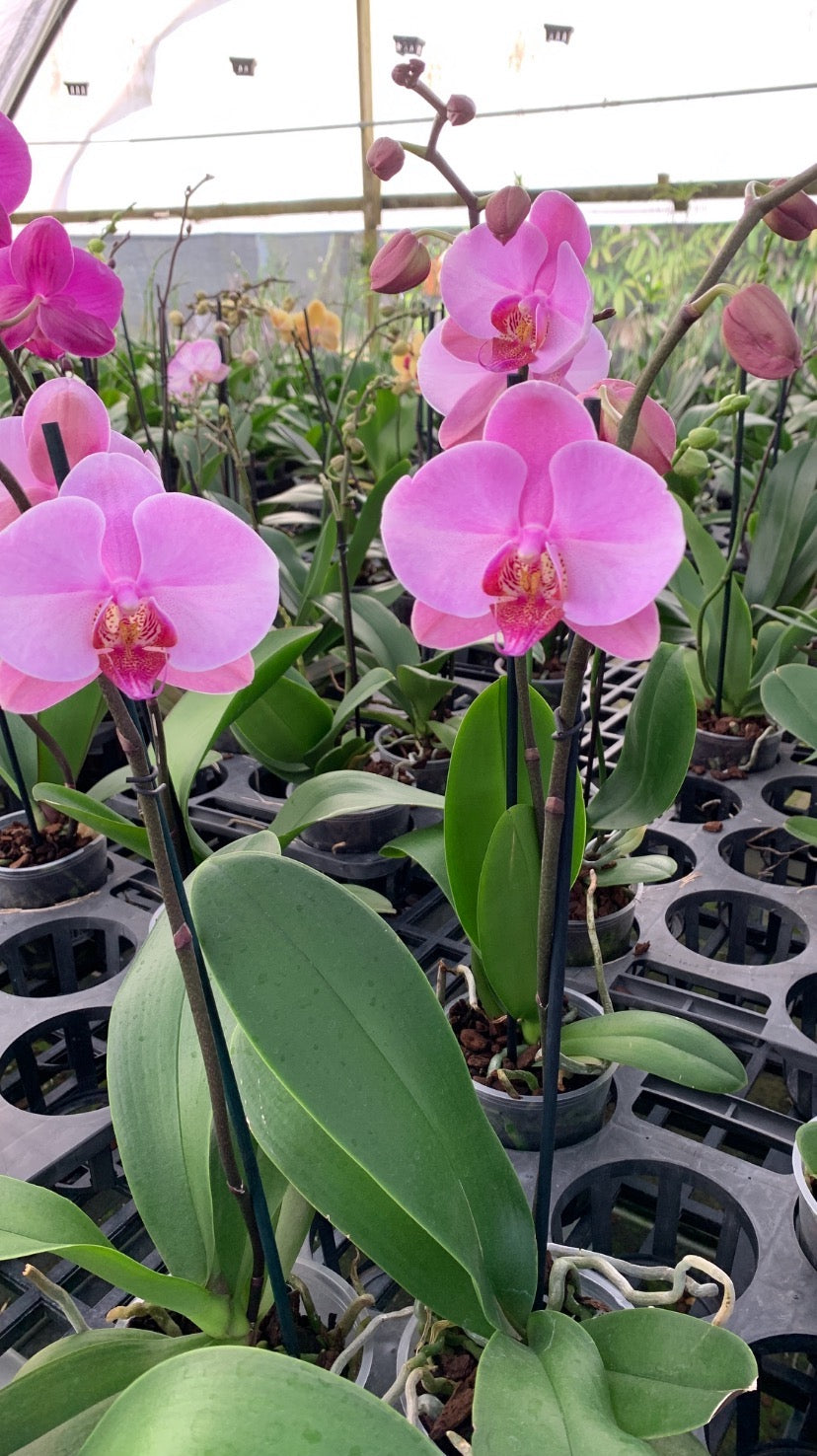This close-up photograph depicts a vibrant scene from a garden nursery or greenhouse. The background features a white, domed canopy supported by a wooden frame, with piping visible at the top likely used for irrigation. The foreground showcases a series of plastic gray planters neatly placed in circular cutouts within plant trays; some trays are empty while others house thriving plants. At the bottom center of the frame, there are small pots with soil containing tall plants characterized by lush, large green leaves and thin brownish-green stems. Blooms of radiant pink flowers, numbering about four or five, dominate the scene. Each flower has six petals—two extending outwards like butterfly wings and three spaced evenly behind. In addition to the primary blooms, the upper left corner of the image features a couple of purple flowers and several pink buds that have yet to unfurl. Other areas reveal a mix of deep yellow and various shades of pink flowers, contributing to the overall diversity and beauty of the greenhouse setting.